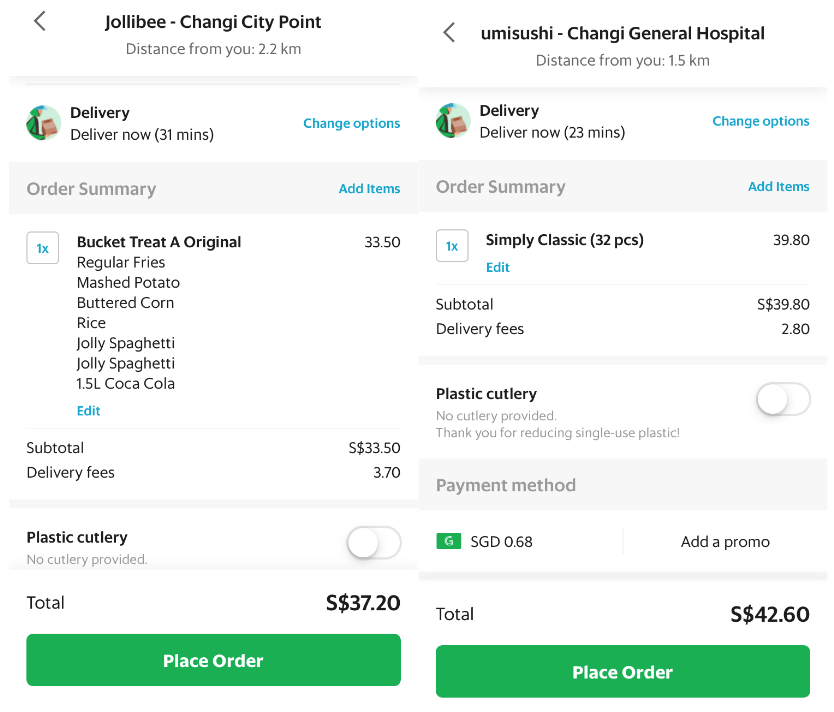In the side-by-side images, the left image displays a phone screen showcasing a food delivery app with an order from Jollibee, located at Changi City Point. The details of the order are explicitly visible: it shows an estimated delivery time of 31 minutes. The ordered items include a Bucket Treat (original), regular fries, mashed potato, buttered corn, rice, and two servings of Jolli Spaghetti along with a 1.5-liter bottle of Coke. The total cost is shown as S$37.20, indicating the currency used is Singapore dollars.

The right image features another food delivery order, this time from Umi Sushi, identified as Changi General Hospital. The delivery time for this order is estimated at 23 minutes. The ordered item listed is "Simply Classic" comprising 32 pieces of sushi. Below this, there is a note about plastic cutlery, indicating 'no cutlery provided.' The image also shows the interface of the app, including a prominent green "Place Order" button at the bottom.

The background and other elements of the app interface give a clear and organized overview of the ongoing food orders from two different locations and their corresponding details.